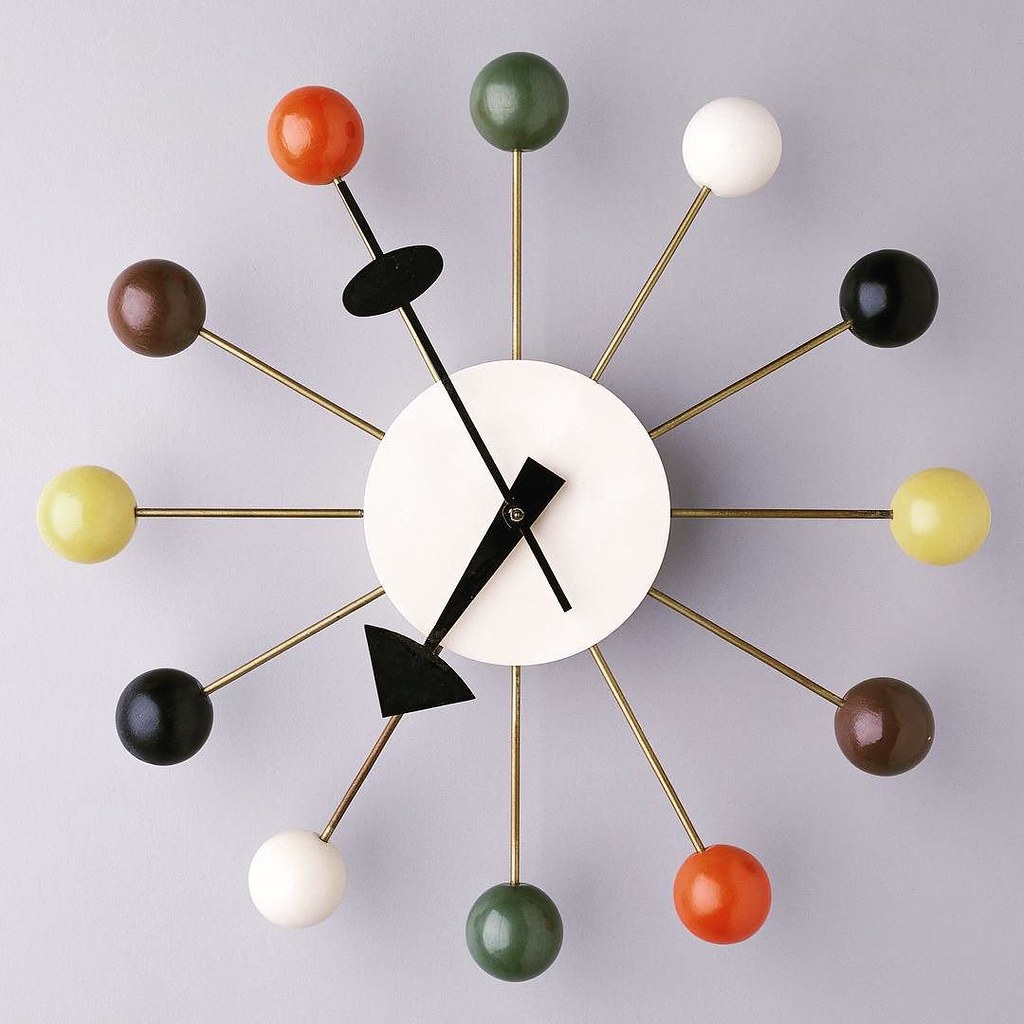This is a wall clock mounted on a pristine white wall. The clock features unique hour markers, each represented by colorful spherical balls attached to golden rods. These rods extend from a central white circle, which serves as the clock's face. The hour markers are designed in a repetitive pattern of colors: starting from the top at 12 o'clock with a green ball, followed by white, black, yellow, brown, and orange, then repeating this sequence.

Two distinct black clock hands mark the time. The minute hand is slender and has an oval shape at its tip, while the hour hand is thicker and ends in a triangular form. The colorful balls, except for the white ones, are glossy, reflecting light and giving a sense of depth and dimension to the clock. Notably, the green ball at 12 o'clock and the other colored balls exhibit this shiny quality, highlighting their vibrancy against the white backdrop.